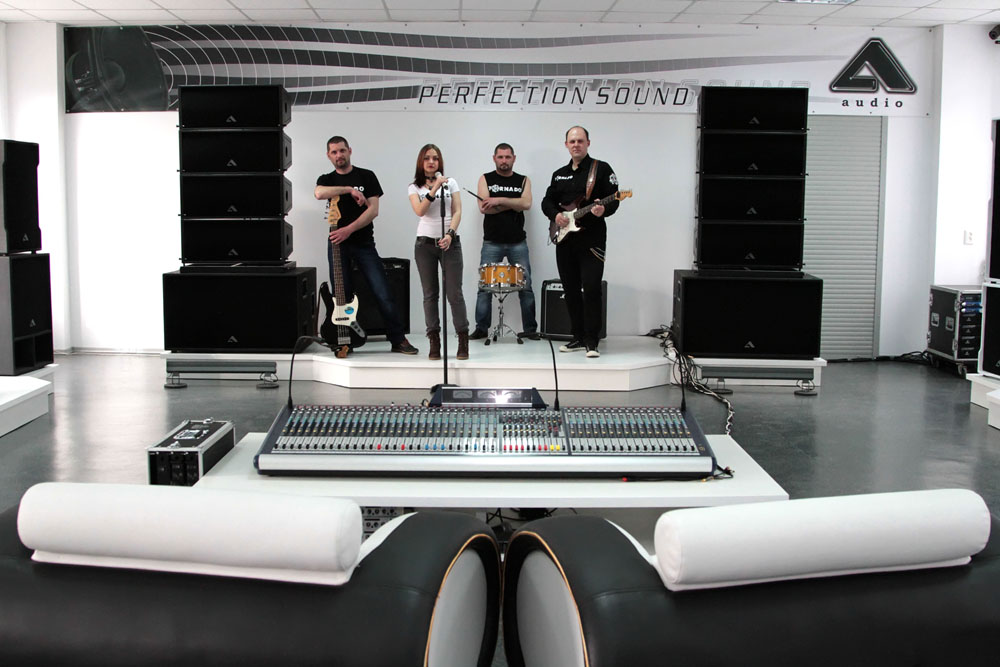The image depicts a professionally posed promotional photo of a rock or pop band situated in a studio. Seen from behind a large soundboard, the viewer is positioned as if they were a sound mixer. The band stands on an elevated white stage, against a backdrop featuring a banner that reads "Perfection Sound Studio" in prominent text at the top. The stage is framed by impressive stacks of speakers—each side boasting a large speaker at the bottom with four smaller ones stacked above it.

From left to right: a man wearing a black t-shirt and jeans holds an electric guitar; next to him, a woman dressed in a white top, khaki trousers, and boots stands at a microphone, suggesting she is the singer. To her right, a bearded man in a black t-shirt with white writing on it and jeans crosses his arms over a single drum and drumstick, looking directly at the camera. The final member, another man with a balding head and a guitar slung around his neck, stands slightly taller than the others and appears to be strumming.

The studio setup features black lighting that shines a white light on the band, enhancing the focus on the musicians. To the extreme sides of the stage, a modern arrangement of music and sound equipment decorates the scene, including a notable guitar case positioned to the left. There is a hint of natural light entering from an external source, possibly a window, underscoring the indoor setting. With its meticulous arrangement and high-quality gear, this image likely serves as a promotional piece for the "Perfection Sound Studio" brand.